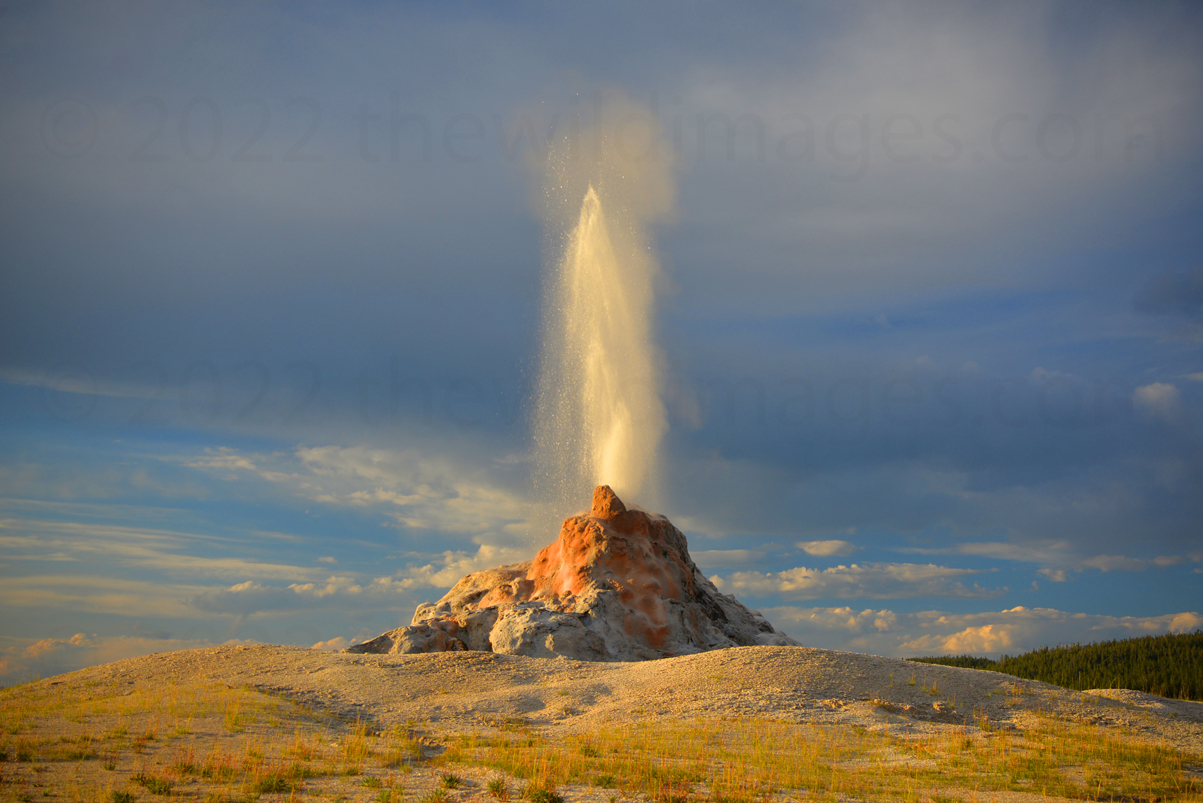The image depicts a dramatic eruption or explosion atop a rugged, rust-and white-colored rocky outcropping, spewing a massive column of white steam high into the sky. The eruption is so intense that debris and steam rise well above the rocky formation itself. The surrounding landscape features a gently rolling valley with sparse patches of green and yellow dry grass interspersed with ashy, light-colored dirt. On the right side of the picture, a distant low hill dotted with green-leaved trees can be seen. The expansive sky dominates most of the upper part of the image, showcasing a mixture of blue hues and various clouds—ranging from white to grayish tones. The image also faintly displays a repeating watermark that reads "copyright 2022, thewildimages.com."